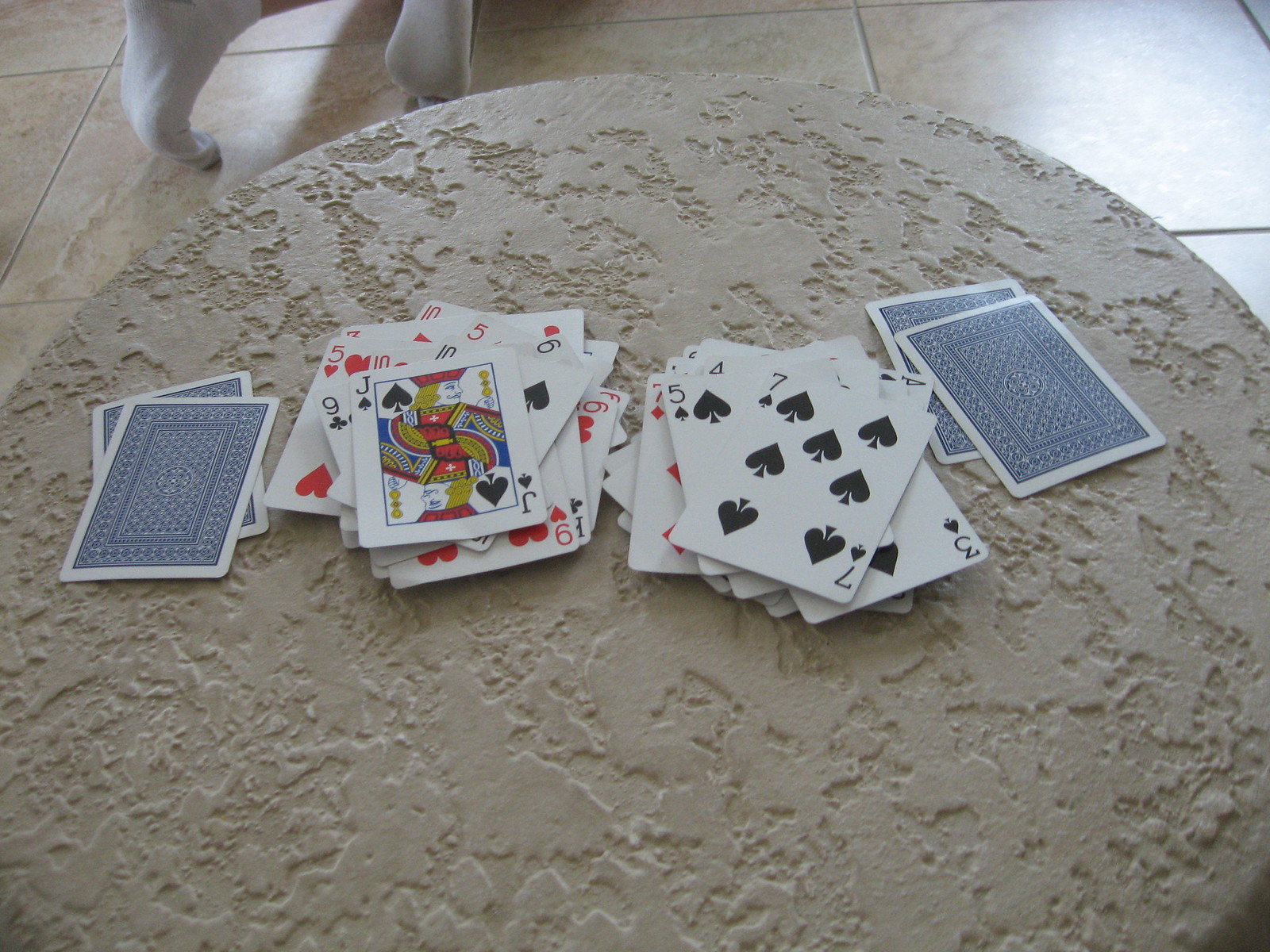The image depicts a footstool-like structure made from what appears to be sheetrock, positioned close to the ground. In the top corner, a pair of feet clad in socks are visible, balanced on their toes in a plank-like position. The focus of the image is four stacks of playing cards arranged in a line. The two outer stacks comprise a few cards each, both face-down with light blue backs featuring an intricate circular pattern. The two inner stacks are face-up, displaying an array of cards. 

The face-up stack just right of the two outer stacks includes a red ten, a red three, a red five, a black six, a five of hearts, a ten of hearts, a ten of spades, a nine of hearts, a king of clubs, a six of hearts, a nine of clubs, a jack of spades, among others. The adjacent face-up stack consists of a seven of spades, five of spades, three of spades, a black four, a nine of spades, a nine of clubs, a ten of spades, a jack of spades, and sequentially arranged cards from three to seven in various suits. 

The cards appear to be part of a sorting game, likely a solitaire variation, where the objective is to sequence cards by color and suit. The detail and alignment of the cards suggest active engagement in organizing or playing this classic card game.